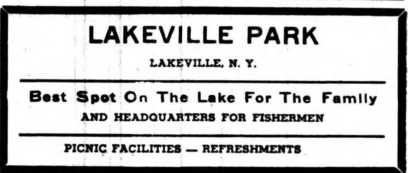The image is a digital screenshot of a vintage advertisement, appearing as a white rectangle with a thick black border. The advertisement, which looks worn and possibly copied from an old magazine or newspaper, features black text that reads:

- At the top: "Lakeville Park"
- Beneath that, in smaller font: "Lakeville, New York"
- Below that, separated by a thin black line: "Best spot on the lake for the family and headquarters for fishermen."
- Followed by another thin black line, it says: "Picnic facilities - refreshments."

The overall impression is one of an old, grainy ad, focused on promoting Lakeville Park as a family-friendly and fisherman-friendly spot with amenities like picnic facilities and refreshments.